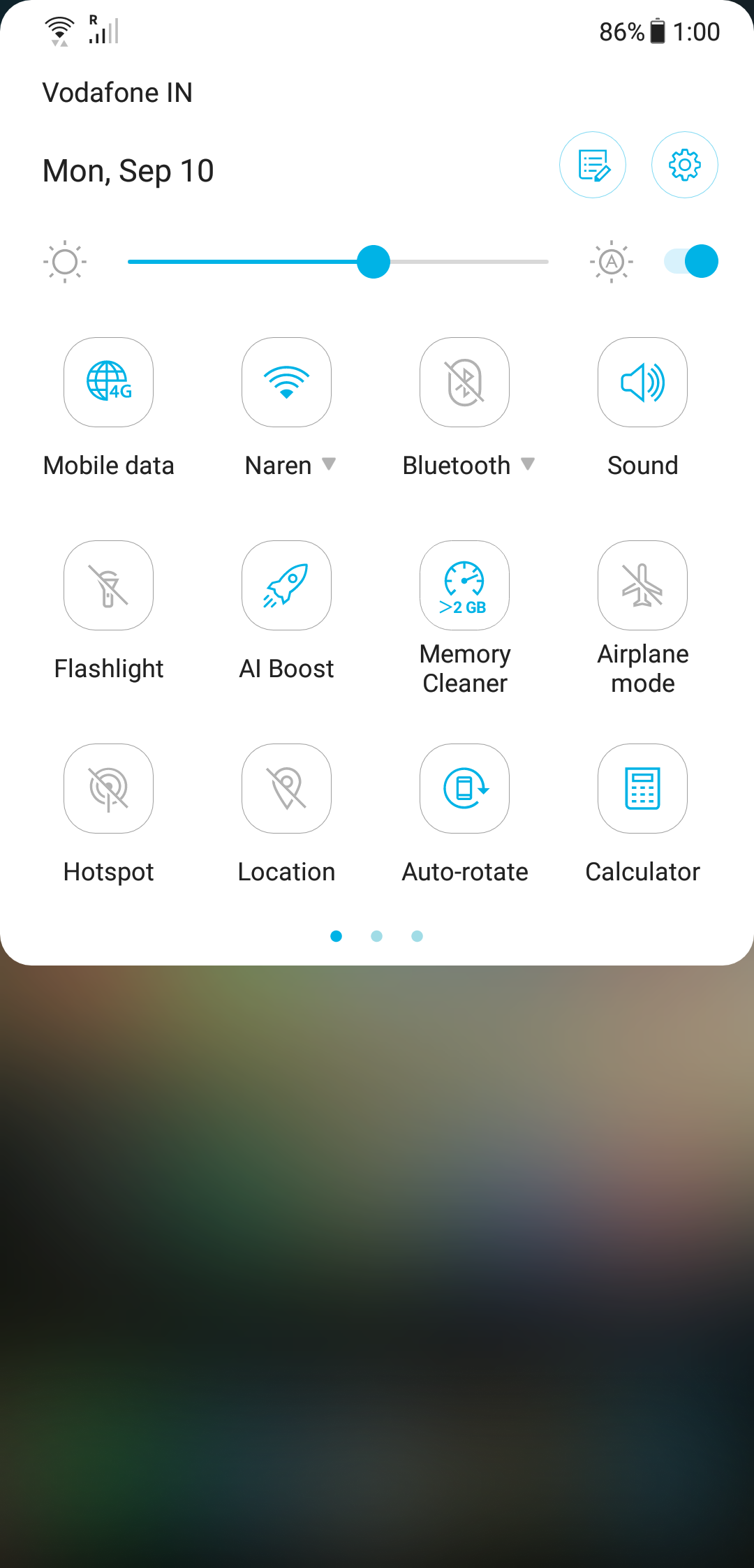This is a detailed screenshot of a smartphone interface. 

**Top Row (Status Bar):**
- **Upper Left Corner:** Displays full Wi-Fi signal and a mobile call signal with 3 out of 5 bars. Above the call signal, there's a capital letter "R" indicating roaming.
- **Upper Right Corner:** Shows the battery level at 86%, and the time is displayed as 1:00.

**Second Row:**
- **Upper Left Corner:** Displays the network provider name "Vodafone" (V-O-D-A-F-O-N-E) and the region "IN" (India) in capital letters. 
- **Center:** Displays the date formatted as "Mon, Sep 10."
- **Upper Right Corner:** Features icons for a notepad with a pencil and a cog (likely representing settings or quick action icons).

**Brightness Level:** The screen brightness is adjusted to slightly above half.

**Quick Access Panel (Pulled Down):**
- **First Row (Left to Right):** 
  1. **Mobile Data**
  2. **Narin** (This could be a custom app or setting specific to the device)
  3. **Bluetooth**
  4. **Sound**

- **Second Row (Left to Right):**
  1. **Flashlight**
  2. **AI Boost**
  3. **Memory Cleaner**
  4. **Airplane Mode**

- **Third Row (Left to Right):**
  1. **Hotspot**
  2. **Location**
  3. **Auto-Rotate**
  4. **Calculator**

**Highlighted/Activated Options:**
- Mobile Data
- Narin
- Sound
- AI Boost
- Memory Cleaner
- Auto-Rotate
- Calculator

This screenshot effectively shows a comprehensive overview of the phone's status, including connectivity signals, battery level, time, network provider, date, essential quick settings, and the current brightness level.